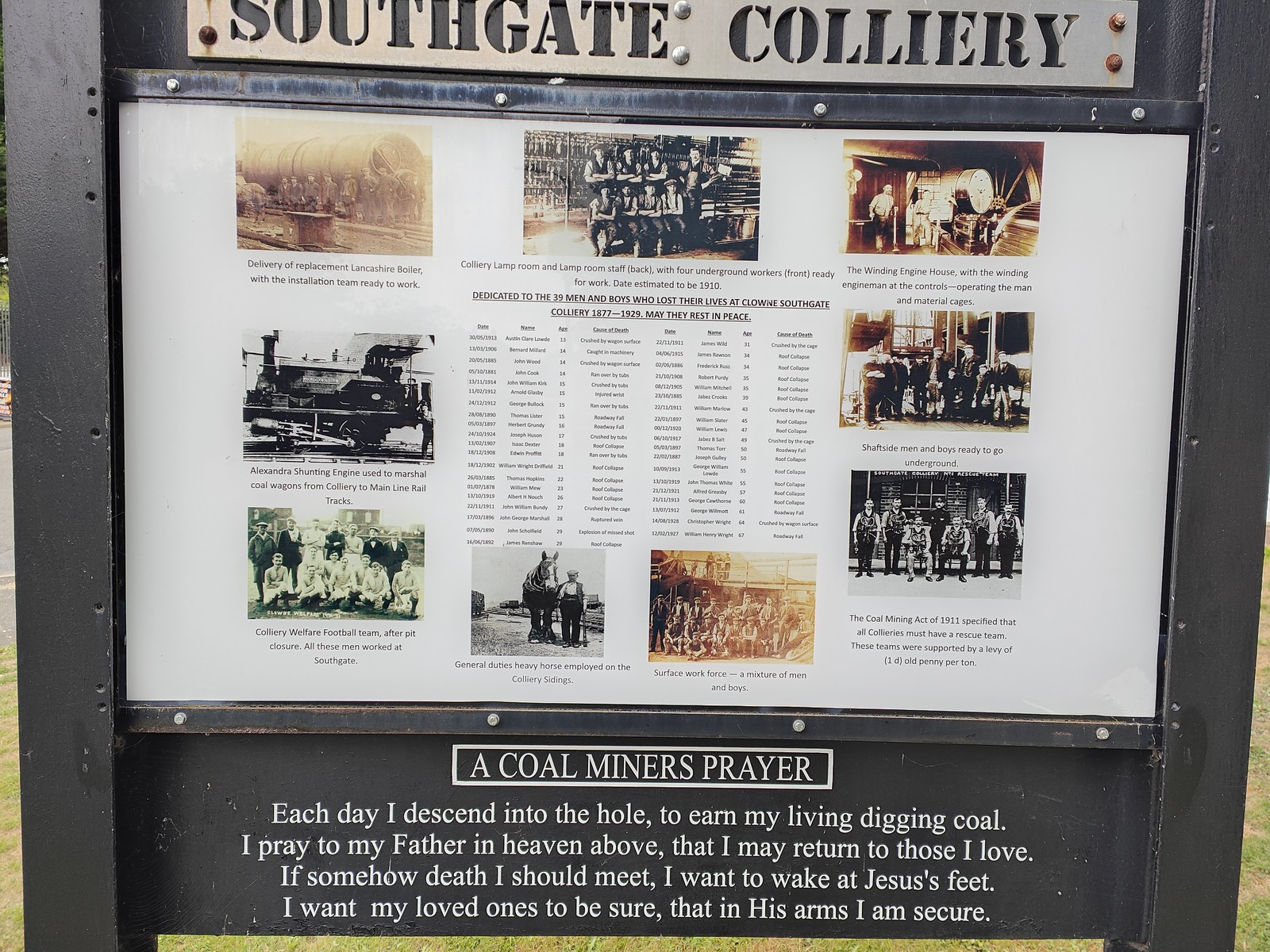The image showcases a detailed informational signboard dedicated to the Southgate Colliery. The signboard is dark gray and features a prominent white plaque at the top, with the words "Southgate Colliery" cut out of metal, revealing the black background of the sign itself. Below this title, there is a detailed plaque containing multiple lines of text and historical photographs. The central portion of the plaque presents nine black-and-white images, including a notable picture of a group of men lined up in two rows, arms crossed and posing for the camera, with the caption indicating they are the Colliery Lamp Room and Lamp Room Staff alongside four underground workers ready for work, dated around 1910. The inscription dedicates the plaque to the 39 men and boys who lost their lives at Clown Southgate Colliery between 1877 and 1929. Underneath these historical details and pictures, the sign concludes with a Coal Miner’s Prayer, reading, "Each day I descend into the hole to earn my living digging coal. I pray to my Father in heaven above that I may return to those I love. If somehow death I should meet, I want to wake at Jesus' feet. I want my loved ones to be sure that in His arms I am secure."